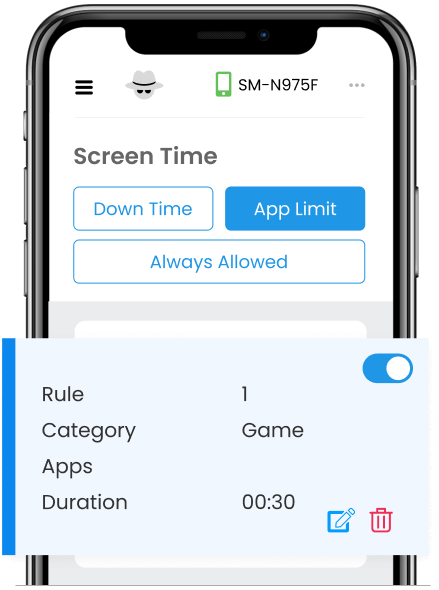The image depicts a vertically-oriented smartphone interface, centered around screen time management features on an Android device. Starting from the top, there is an outlined illustration of an Android figure in black. At the topmost part of the screen, a black bar houses a small black camera icon with a blue dot to the right indicating activation. 

Below this, a set of status icons are aligned. On the far left, there are three stacked horizontal black lines (possibly representing a menu or navigation option). Next to this, there's a cartoon avatar of a figure in a gray cowboy hat with sunglasses, featuring a black ribbon around the hat's base. 

To the right of the avatar, a green icon symbolizing an Android device is visible. Adjacent to this, large black text reads "SM-N975F", identifying the specific phone model. Towards the far right of the status icons, there are three medium-sized gray dots arranged vertically.

Further down, a thin gray line spans horizontally beneath these icons. The text below this line reads "Screen time" in gray letters. Subsequent to this heading is a selectable blue-bordered box with the word "Downtime" written in blue letters against a white background.

To the right of this, another box is present, this time filled with blue and the text "App limit" in white letters. Beneath these options is a long blue-bordered box labeled "Always allowed" in blue letters on a white backdrop.

The lower section of the screen transitions into a gray area with a white box, partially covered by a faint blue bar extending vertically. This box contains detailed statistics, featuring text aligned to the left side: "Rule", "Category", "Apps", and "Duration". To the right of this text, the numeral "1" is displayed.

Below this section, the category "Game" is indicated, followed by a duration of "00:30". In the upper right corner of the pale blue box, an active toggle switch is displayed, with the white circle inside a blue background indicating it is switched on. 

In the lower right corner, a small, pale blue square contains a pencil icon pointed towards the lower left, signifying an edit function. On the far right corner, a red trash can icon denotes the delete option.